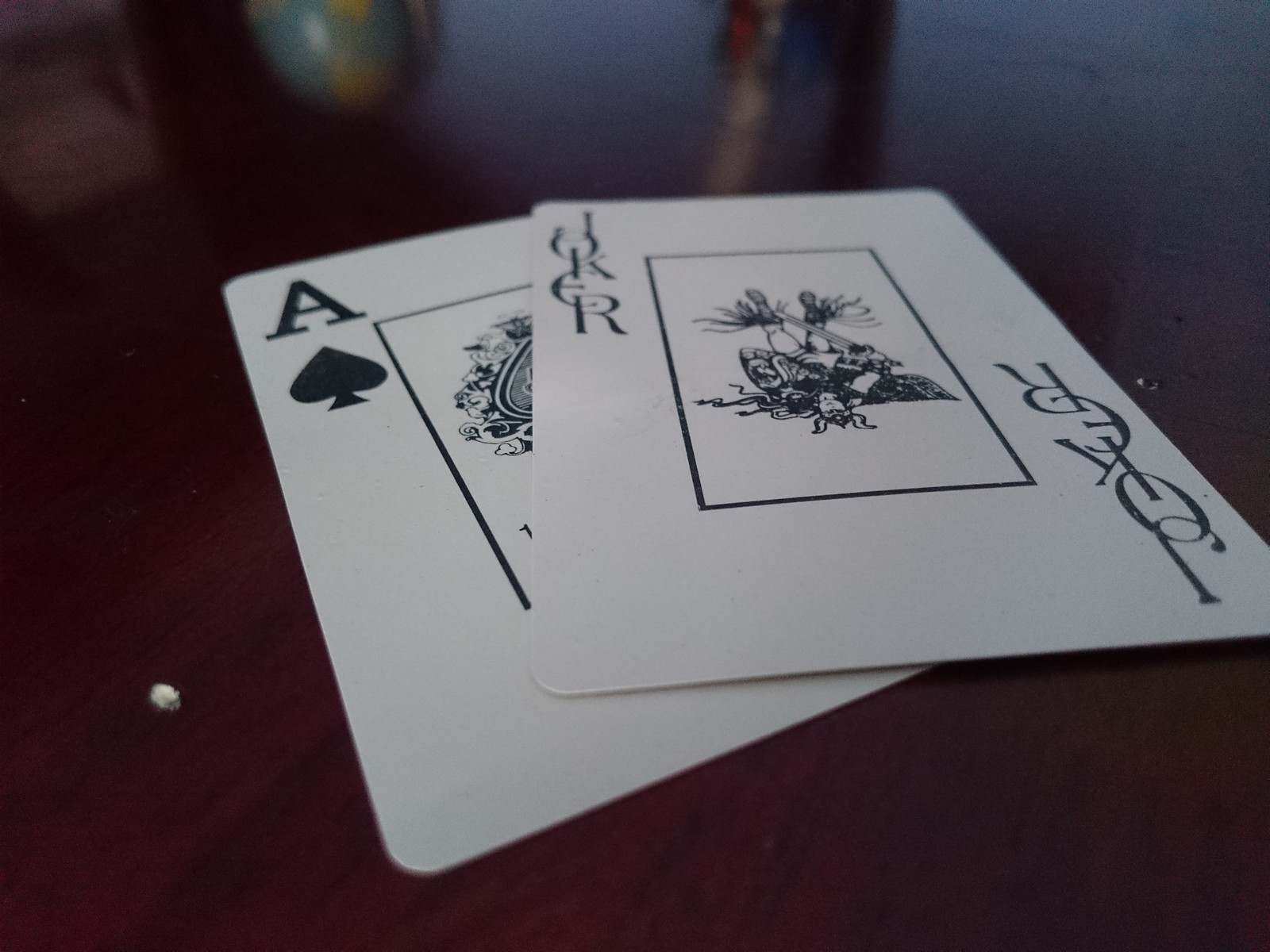A rectangular photograph showcases two horizontal playing cards resting on a dark, shiny wooden table. The bottom card is the ace of spades, identifiable by the capital 'A' in the left-hand corner, beneath which sits a spade symbol—an upside-down heart with a flared stem resembling a tree stump. This ace card also features a partial, decorative black border, though much of it is obscured by the card resting on top. 

The overlaying card is a joker, positioned at an angle and covering roughly half of the ace of spades. The joker card displays the word "JOKER" vertically along the top left edge, with each letter staggered slightly to the left or right. On the opposite side, the right-hand bottom edge, "JOKER" is spelled in reverse, appearing upside down. The central image on the joker card depicts an upside-down jester, showing his white pants, boots with strings flying off, and cape. His face, painted white with snake-like tendrils extending from his head, adds to the card's whimsical aesthetic.

In the background, the table's polished surface reflects various objects, including a globe in the upper left-hand corner. Other indistinct items are also mirrored on either side of the globe, adding a layer of subtle complexity to the scene.